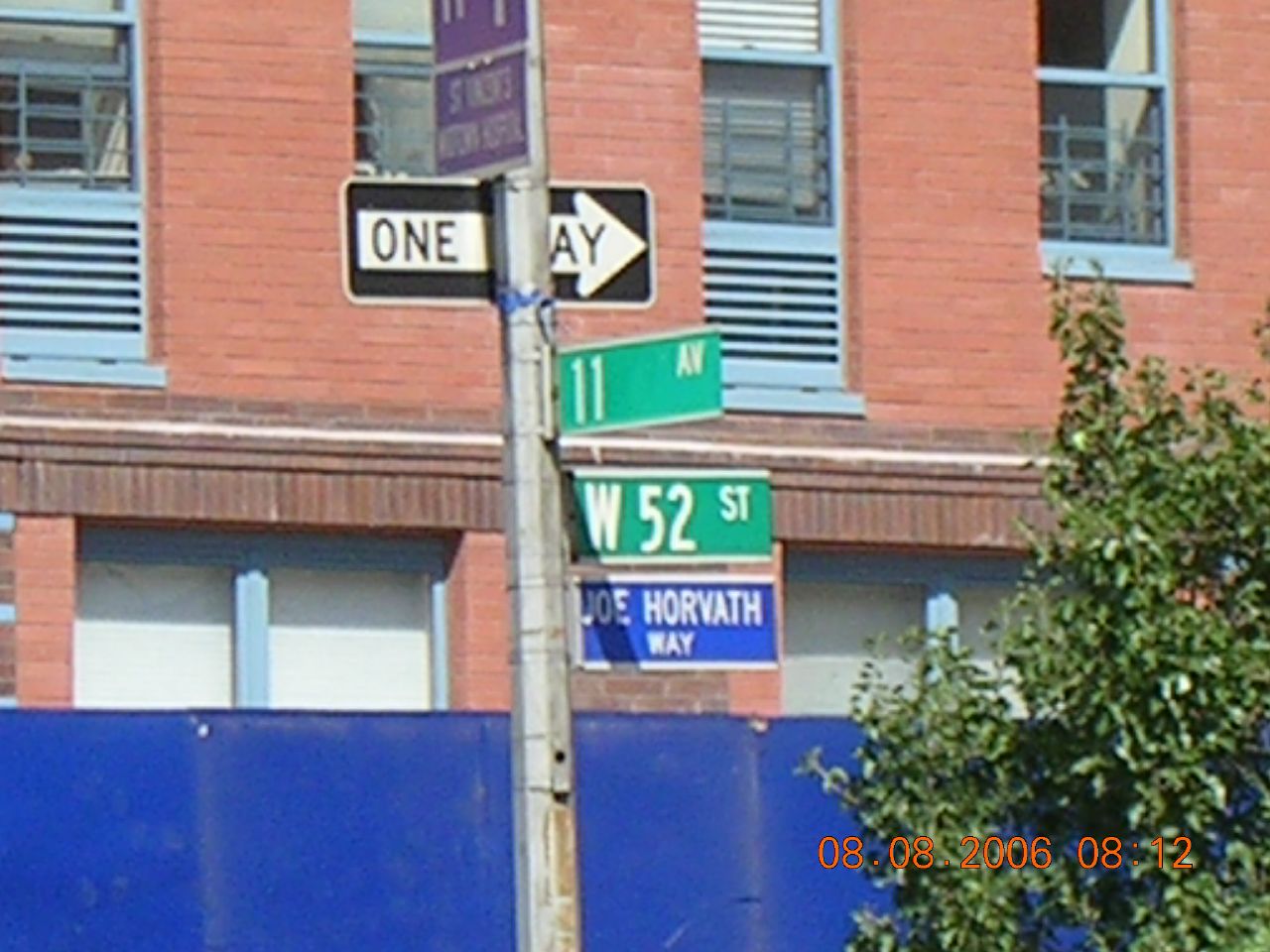The image, dated August 8, 2006, at 8:12 a.m., is set outdoors in front of a brick building that appears to be an apartment complex or housing unit with traditional brick coloring. The building features several gray-framed windows, some with venting at the bottom. The lower level of the building has gray wood boarding with white detailing behind it. In front of the building, there's a gray metal pole displaying multiple street signs: "11th Ave," "W 52nd Street," "Joe Horvath Way," and a "One Way" indicator. Adjacent to the pole stands a tall green tree with small leaves. A large blue fence or tarp, possibly a dumpster, runs along the bottom of the image, partly obscured by the building. A green plant or shrub is visible in the bottom right corner. The photo captures a mix of urban elements like street signs and natural features against the backdrop of the brick building.